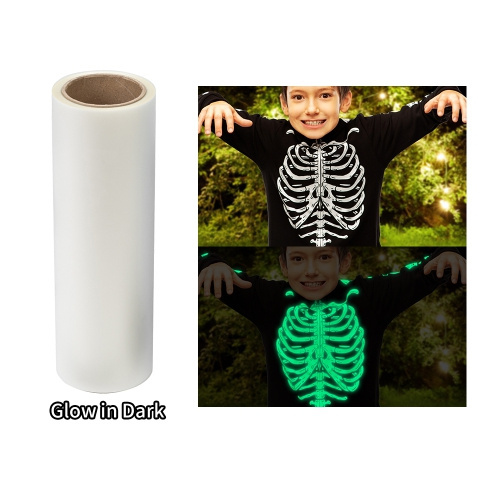The image appears to be an advertisement featuring a glow-in-the-dark product. On the left side, there's a roll of white material, possibly tape, wrapped around a cardboard tube, with the words "glow in the dark" written below it in black outline with white font. On the right side, two images are stacked vertically. The top image shows a happy little boy with his arms raised in a playful, scary gesture, wearing a black sweater with printed skeleton bones depicting a human ribcage and spine. The background features green trees with string lights and daylight filtering through. The bottom image is a darkened version of the same scene, where the skeleton bones on the boy's sweater and some tape on his sleeves glow bright green, emphasizing the product's glow-in-the-dark capability. The whole scene is set against a translucent background, and the boy appears joyful with a big smile and visible teeth, showcasing how the product functions in both light and dark conditions.